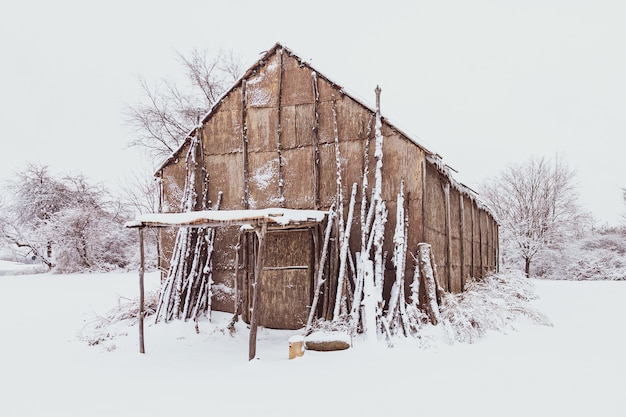This image captures an Indian barn, crafted from birch bark and stretching approximately 20 feet tall. The barn, often termed a "birch bark barn," features a small awning over a porch at one end. Several wooden poles and an assortment of branches are visibly propped against the structure. The barn is enveloped in snow, with at least a couple inches blanketing its surface, accentuated by numerous icicles hanging from the roof.

Surrounding the barn, there is an expanse of white snow, indicative of a recent or impending snowfall, under a stark white sky. Alongside the barn lies a line of small bushes, heavily laden with snow. The background is dominated by a field of snow, dotted with scrubby bushes and small, branchy trees, all equally covered in snow. The barn's material, which some might interpret as straw or hastily assembled plywood, adds to its rustic charm. The colors in the scene are largely muted, dominated by browns from the barn and white from the snow, creating a tranquil yet stark winter landscape.